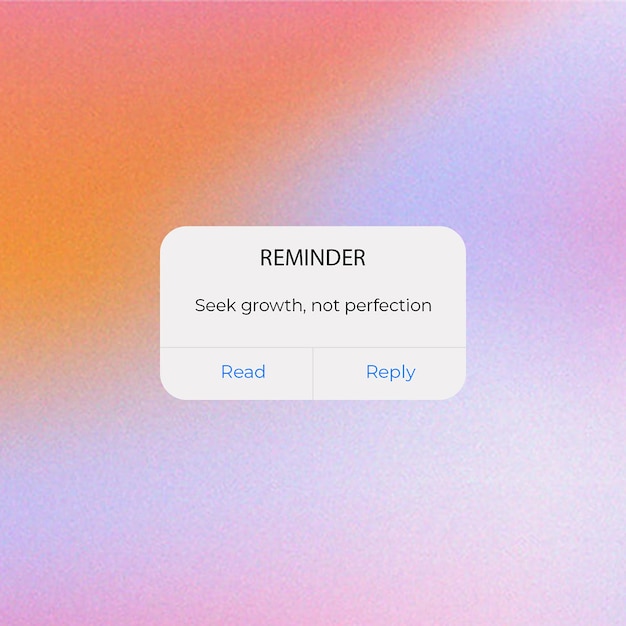The background features a gradient of colors starting from a rich orange on the left, transitioning into a soft lilac or light purple, then melding into pink and white shades. At the bottom, there are two bands of very light pink that extend from the left to the right, with the right-hand side blending back into white and then pink again, merging subtly with the purple hues above.

Centrally located is a light gray rectangle, reminiscent of the color used in cement that holds red bricks together in a wall. On this rectangle, in bold black capital letters, are the words "REMINDER." Below, in smaller font, it reads, "Z-Crow, not perfection." A thin gray line runs horizontally across the bottom of the rectangle, bifurcating it and leading to two buttons. The button on the left is blue and labeled "Read," while the button on the right is also blue and labeled "Reply."